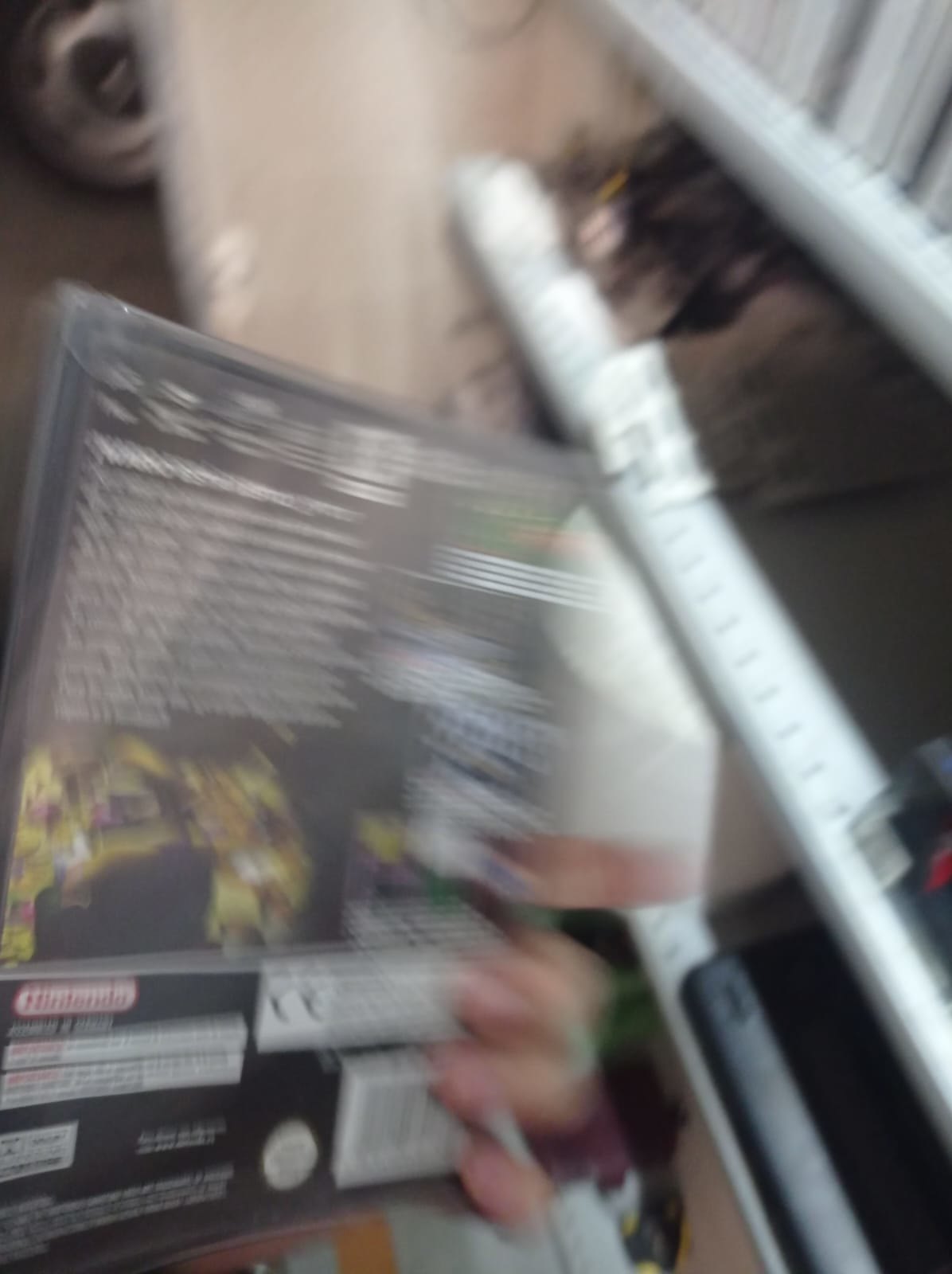In this slightly blurry photograph taken from above, various objects are scattered against a black background. At the bottom left, the edge of a CD case with white writing is visible, encased in its clear plastic cover. The bottom of the image features several white rectangles adorned with black text. From the bottom right, a white metal piece with holes, possibly part of a structure, protrudes and extends into a piece of plywood, with a black piece of plastic affixed near the base. Another similar white metal rod is positioned slightly above and to the right of the first. Additionally, a vertical white line traverses the upper right corner, adding an element of linear contrast to the composition.